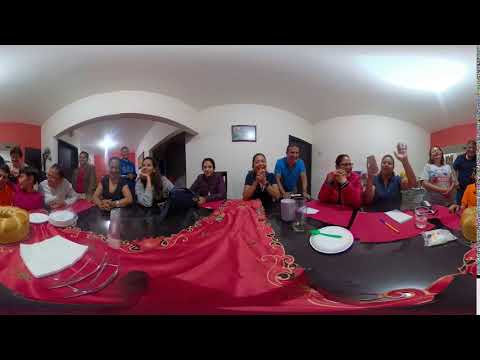The image depicts an indoor scene with approximately 10 to 15 people gathered around a large, brown wooden dinner table. The table is adorned with an ornate red tablecloth featuring intricate gold and black accents along the seams. White dishes and red napkins are arranged in front of the guests, who also have glasses on the table. A cake or bread is present among the settings, suggesting a shared meal or celebration. The background reveals a room with predominantly white, curved walls, and a ceiling that reflects light, creating a bright atmosphere. Additionally, there are sections of the wall painted red, contributing to the room's warmth. On the left-hand side of the image, a white archway is visible, enhancing the architectural detail of the setting. The overall ambience suggests a gathering characterized by a blend of casual and formal elements.